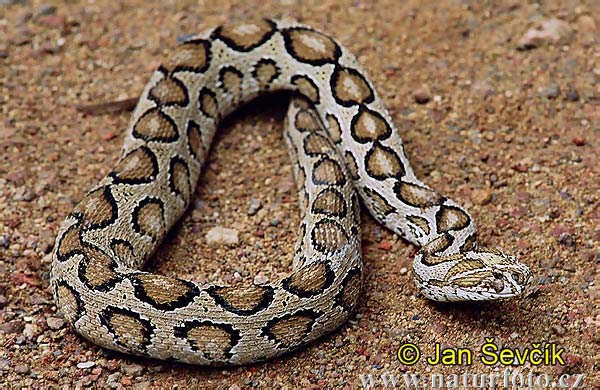This detailed image features a coiled snake, likely a rattlesnake, resting on a rocky, pebble-strewn ground that is predominantly brown. The snake's body showcases a striking pattern of light brown and dark brown patches, interspersed with messy, black-edged circular markings filled with white. Its coloration varies from gray to hues of brown, blending seamlessly with the earthy backdrop. The snake's head is positioned towards the right side of the frame, and although its tail is not fully visible, portions of it can be seen under its coiled body. Notably, the photograph's close-up nature captures intricate details and textures, highlighting the snake's robust build. The image is bright and well-defined, bearing the photographer's signature at the bottom right in yellow font, "Jansevcik," followed by the website "www.naturephoto.easy" in white font.